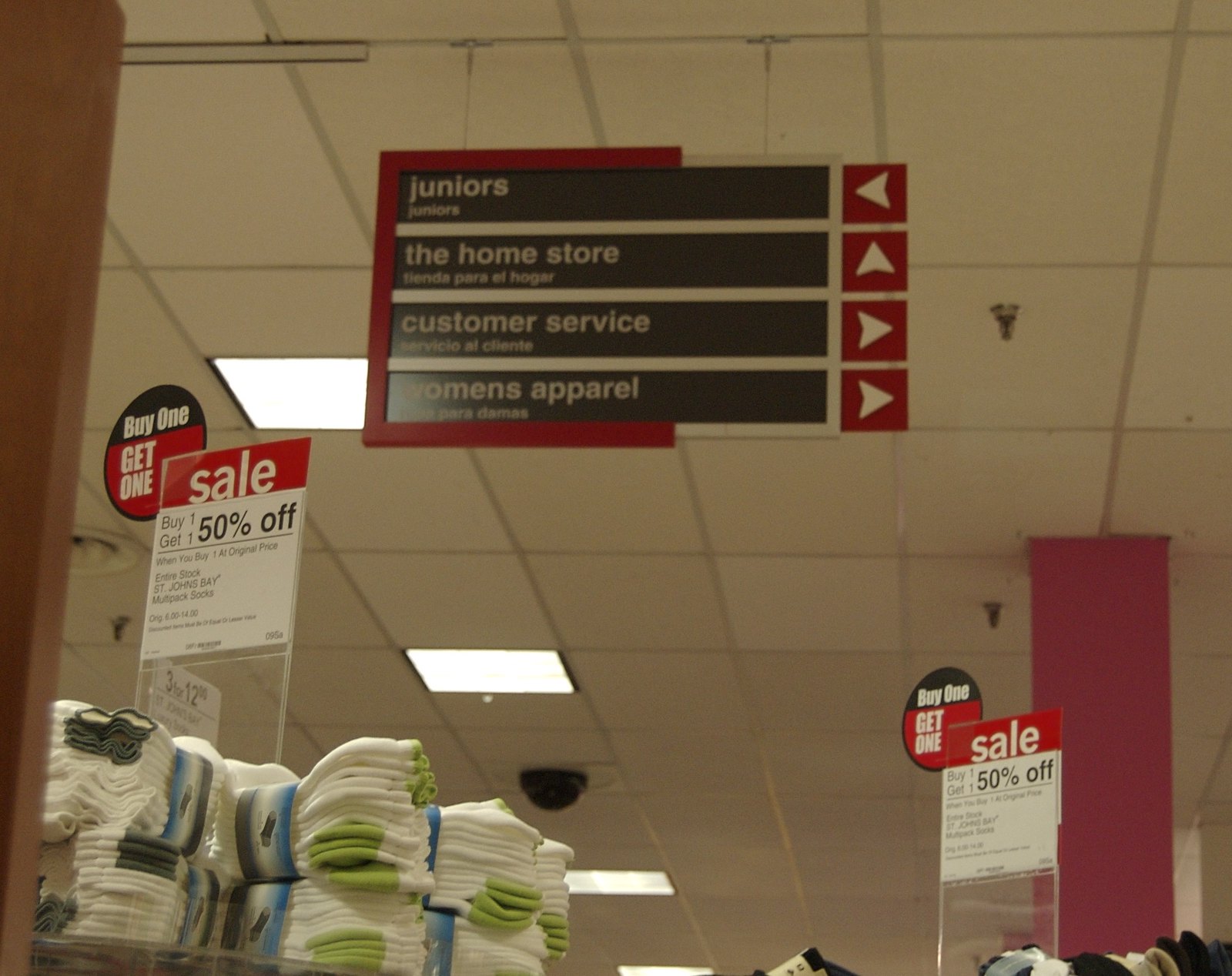The image captures an interior aisle of a Target store, with the photograph taken from an angle slightly above the top shelf of a display, just understandably wider than tall. The ceiling is prominently featured, showcasing a pattern of white tiles forming various small squares, some of which contain rectangular, bright white lights. Centrally, there is a hanging rectangular sign suspended by two wires from the ceiling. The sign is red, gray, and black, and includes directional arrows to the right (left, up, right, right) with corresponding labels in off-white against black bars on the left. The labels indicate the sections: Juniors, the Home Store, Customer Service, and Women's Apparel. At the lower portion of the image, there are additional signs stating "Sale, Buy 1 Get 1, 50% off." On the left side of the display below these signs, there appears to be a stack of socks, predominantly white with occasional dark black and mossy green accents.